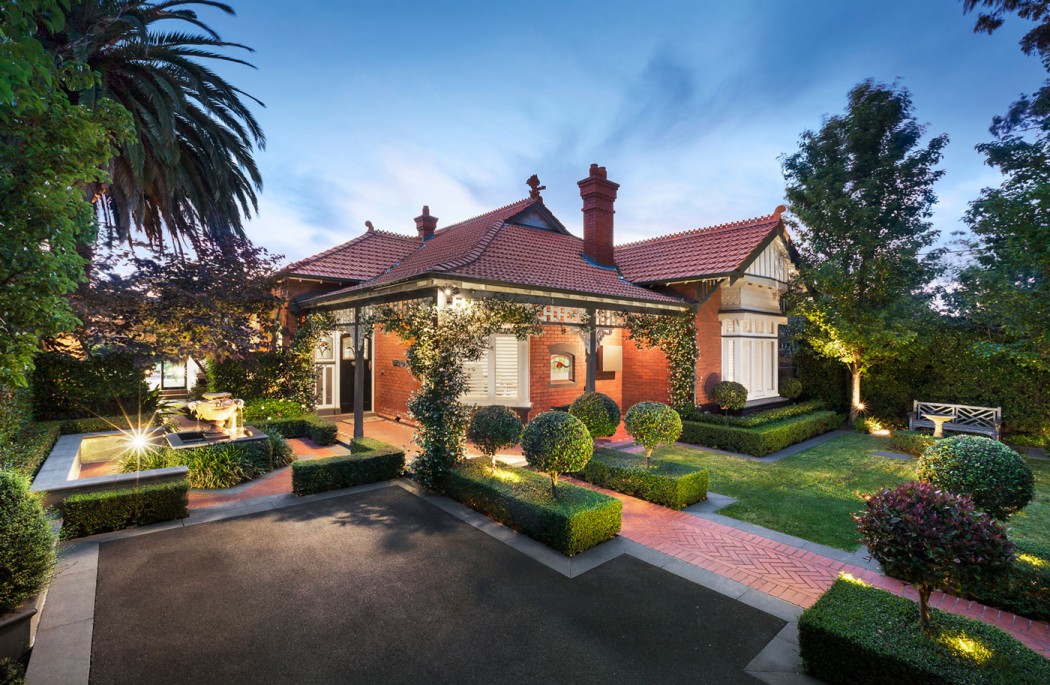This image depicts a beautifully maintained, computer-generated residential house that exudes an air of meticulous care and suburban charm. The house, painted a bright red with contrasting white-framed windows, features a darker red roof adorned with a chimney, adding a touch of rustic elegance. The architectural design of the roof is varied, showcasing multiple pitches and points indicative of a ranch-style home. An overhang porch, supported by gray wooden posts entwined with lush green vines, extends from the front entrance along the side of the house, further enhancing its picturesque appeal.

Surrounding the house are various well-manicured landscaping elements. On the right side, a neatly trimmed lawn hosts a wooden bench and some strategically placed lights, contributing to the cozy atmosphere. Taller green-leafed trees and precisely shaped square bushes, alongside a vibrant palm tree, add depth and variance to the garden’s design. The left side features a charming fountain encircled by green bushes, with a conspicuous bush flaunting red and pink flowers at the bottom right corner. The entire scene is illuminated, accentuating the perfection of each detail.

A red brick paver sidewalk, bordered by gray stone tiles, leads up to the black entrance door, integrating seamlessly into the stunningly maintained concrete driveway. The clear blue sky with scattered white clouds in the background further emphasizes the idyllic and almost surreal quality of this scene, making it hard to distinguish whether this immaculate house and its surroundings are a digital artwork or a real-life masterpiece.